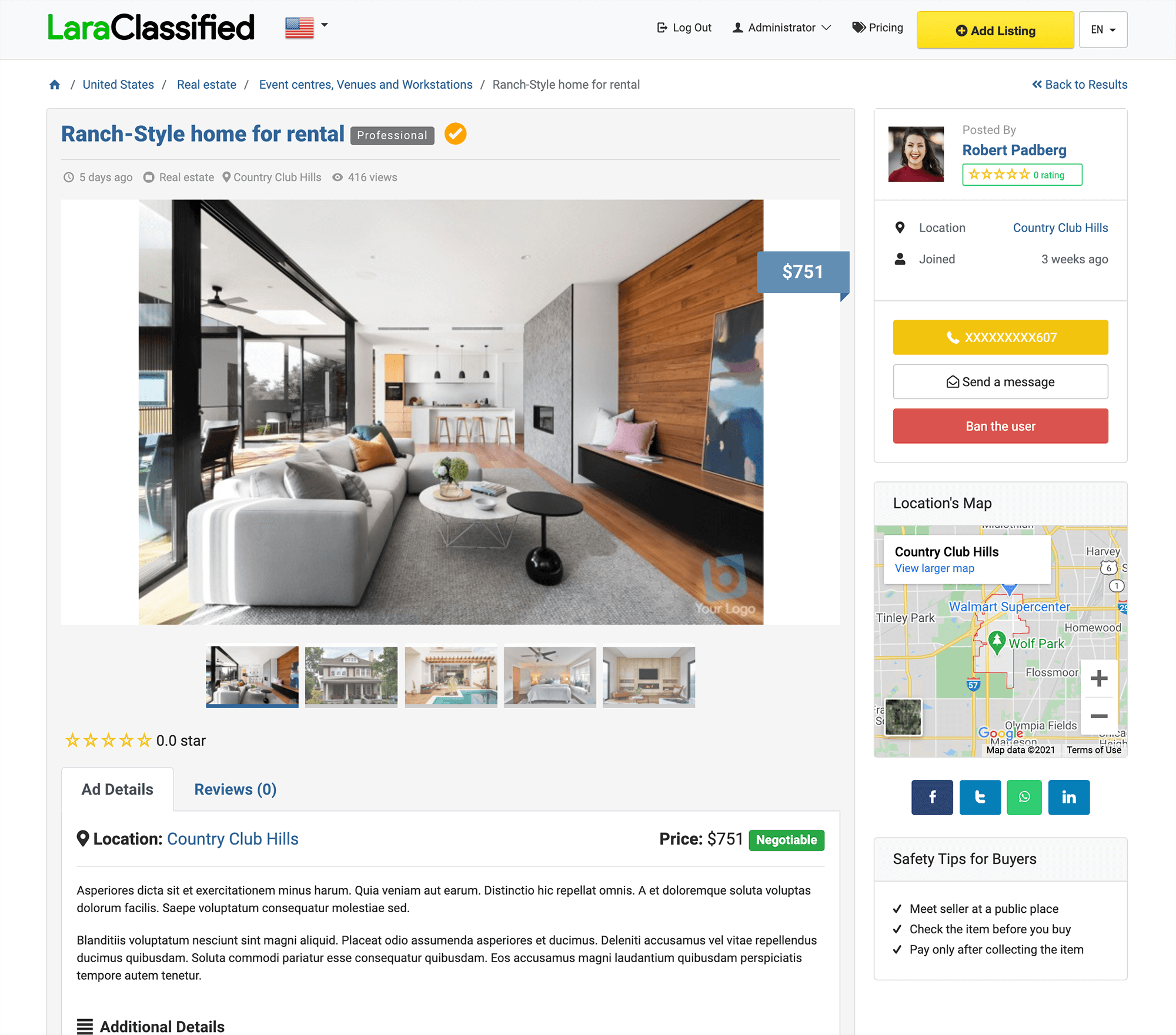This image is a cropped screenshot of a page from a classifieds website named "LaraClassified." The logo is positioned in the top left corner, with "Lara" written in green and "classified" in black, forming a single-word brand name. Adjacent to the logo is an American flag icon followed by a drop-down menu indicating that the language is set to English.

On the far right, the header features icons for logout, administrator access, and pricing, accompanied by a prominent yellow button labeled "Add Listing." There is also a smaller drop-down menu next to this button, which is set to English.

At the top section of the page, there is a prominent blue box with a listing titled "Ranch Style Home for Rental." This box includes a small gray rectangle at the top-left corner inscribed with the word "Professional" in white font, and a yellow circle with a white check mark, signifying a verified post. Below this, details such as the posting date, category, location, and the number of views are displayed. 

The visual content of the listing includes property thumbnails, with a single large thumbnail prominently featured. To the right of this main image, a blue banner displays the rental price of $751. A horizontal row of additional thumbnails appears below the main image, where the first thumbnail matches the enlarged view while others are grayed out but clickable for enlargement.

Further down in the left section, there is a star rating system. Below this, there are two tabs: "Add Details," which is currently selected, showing detailed descriptions of the house, and a "Reviews" tab. Reiterating the price, the top-right section of this description box mentions $751, paired with a green box indicating that the price is negotiable.

On the right side of the listing, information about the poster is provided, including their location, member duration, contact number, and options to send a message or ban the user, indicating that this page is part of the admin panel.